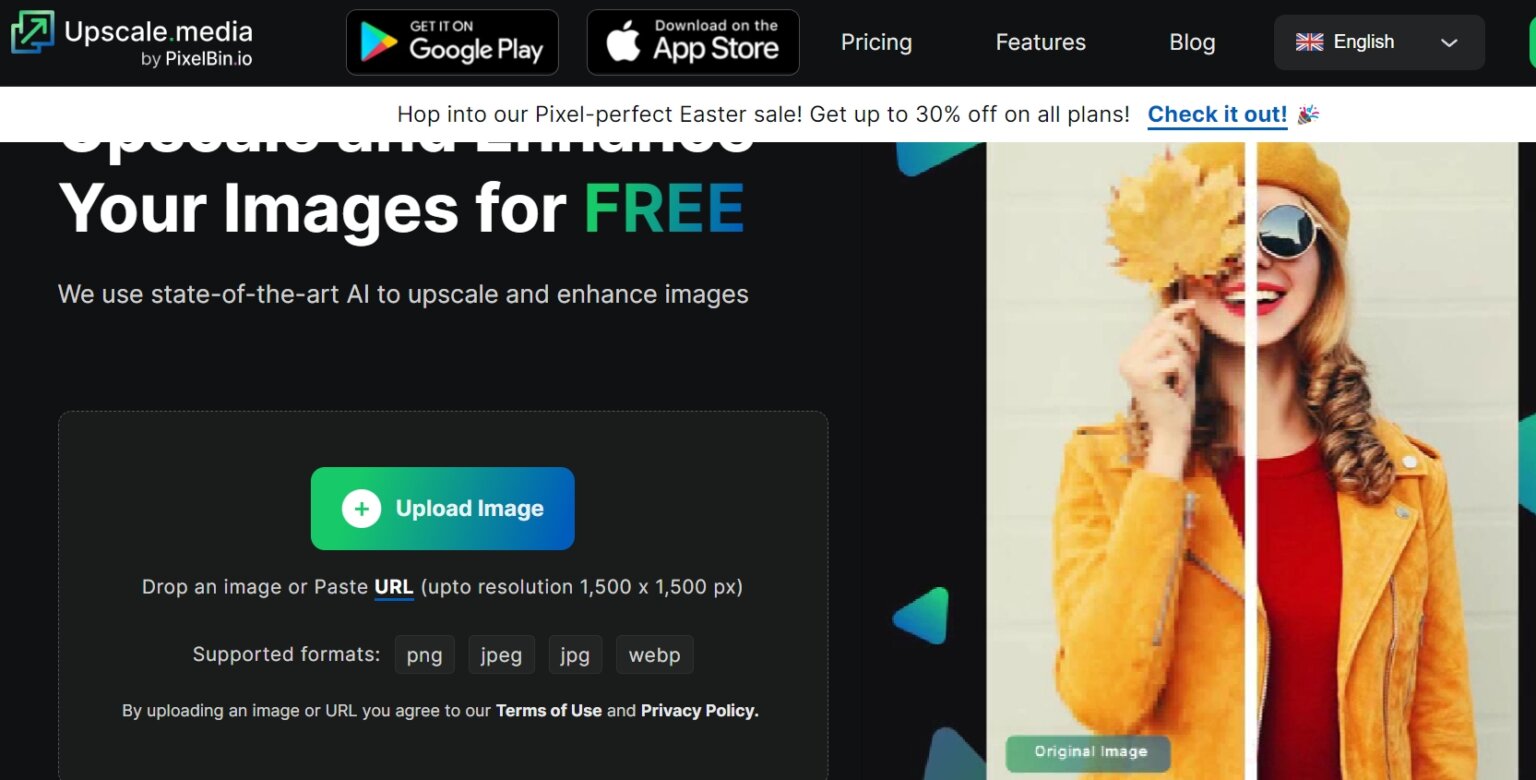This image captures the homepage of a high-end media enhancement website. The logo, positioned in the top left corner, features two interlocking squares with an arrow through them, emphasizing precision and progression. Next to the logo are prominent buttons for downloading the app: "Get it from Google Play" and "Download on the App Store." In the top right corner, the language is set to English, catering to an international audience.

Dominating the right half of the page is a striking image of a woman in an orange coat, wearing glasses and playfully holding a leaf over one eye, injecting a sense of creativity and natural beauty into the site. Just below the main navigation, a vibrant banner advertises a "30% off" promotion with the call to action: "Check It Out."

Immediately below the banner is a bold header reading "Enhance Your Images for Free," highlighting the primary service offered. A subheading further elaborates: "We Use State-of-the-Art AI to Upscale and Enhance Images," assuring users of the advanced technology behind the service. This section features a large, eye-catching blue and green button labeled "Upload Images," inviting users to get started easily. Additionally, the site offers an option to "Drop an Image or Paste URL" for seamless uploads.

At the very bottom, the site lists the supported formats, ensuring users are well-informed before they begin their image enhancement journey. The layout is clean and professional, with a clear emphasis on usability and innovation.